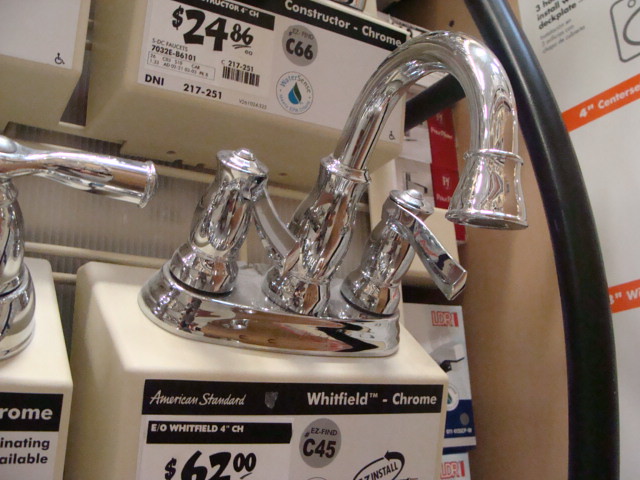This image captures a detailed display of bathroom faucets in a home improvement superstore, likely Lowe's or Home Depot. The focal point is a sleek American Standard Whitefield faucet in chrome, prominently mounted on a cream-colored box attached to a wall. This three-hole faucet features two chrome handles and a central spout, and is priced at $67. Detailing on the box includes black and white stickers with various codes and a price tag. Above this faucet, a Constructor chrome faucet is displayed, priced at $24.86. The scene reveals additional faucets positioned adjacent and above the main focal point, aligned on a shelving unit. The background includes elements like black trim, a blonde wooden board, and unreadable white signage on orange bands, lending context to the store setting. The color scheme comprises silver, black, beige, and white, juxtaposing coordinated displays with functional, aesthetic appeal.